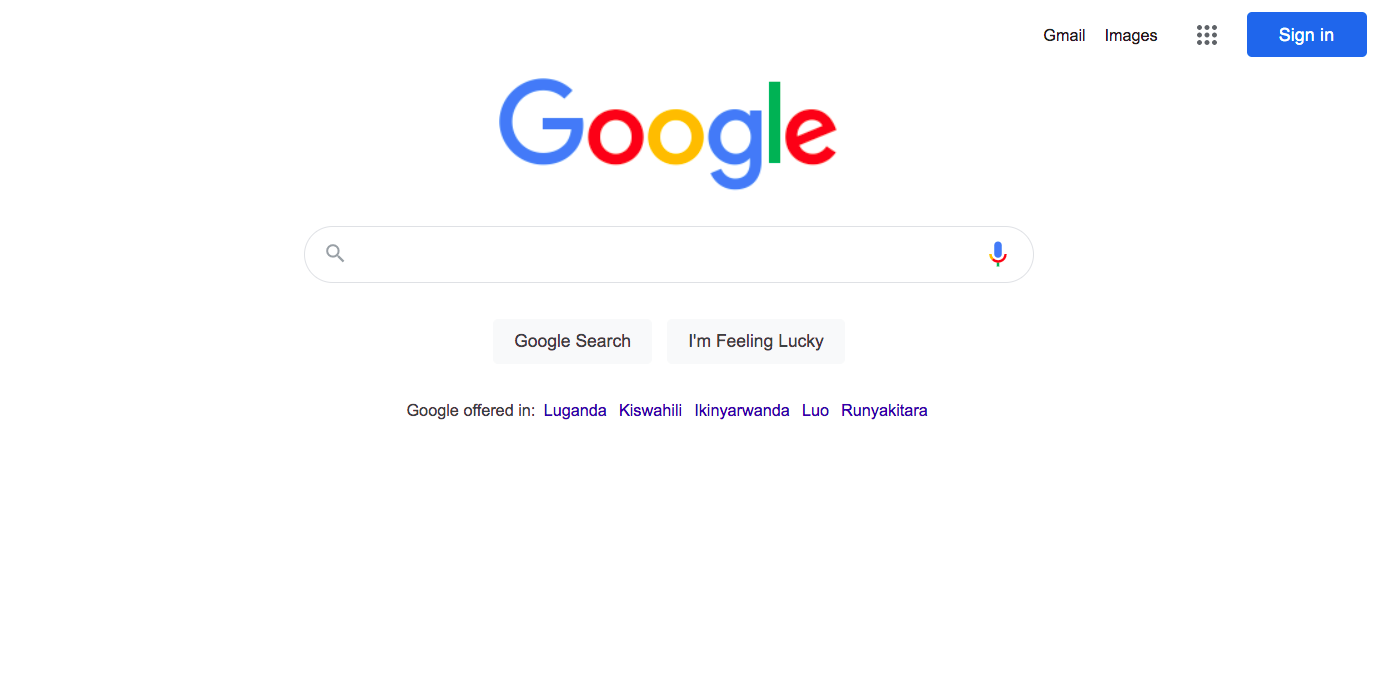The image shows the main Google search page. At the top of the page, there are links to "Gmail" and "Images." The familiar Google logo is prominently displayed, featuring the blue "G," red "o," yellow "o," blue "g," green "l," and red "e" characters. 

Beneath the logo is the main search bar with an oval shape that includes a magnifying glass icon on the left and a microphone icon on the right. Below the search bar, there are two buttons labeled "Google Search" and "I'm Feeling Lucky."

To the right of "Gmail" and "Images," there's a grid icon made up of 9 dots to access Google apps. Additionally, the page offers language options including Lugana, Kiswahili, Etinia, Rwanda, Luau, Lunya, and Kitara, suggesting that the picture might have been taken from a region where these languages are spoken.

There are no visible options for "Sign In" on this particular Google page, and the background includes subtle blue tints, though it didn't trigger any noticeable interaction such as a tingle.